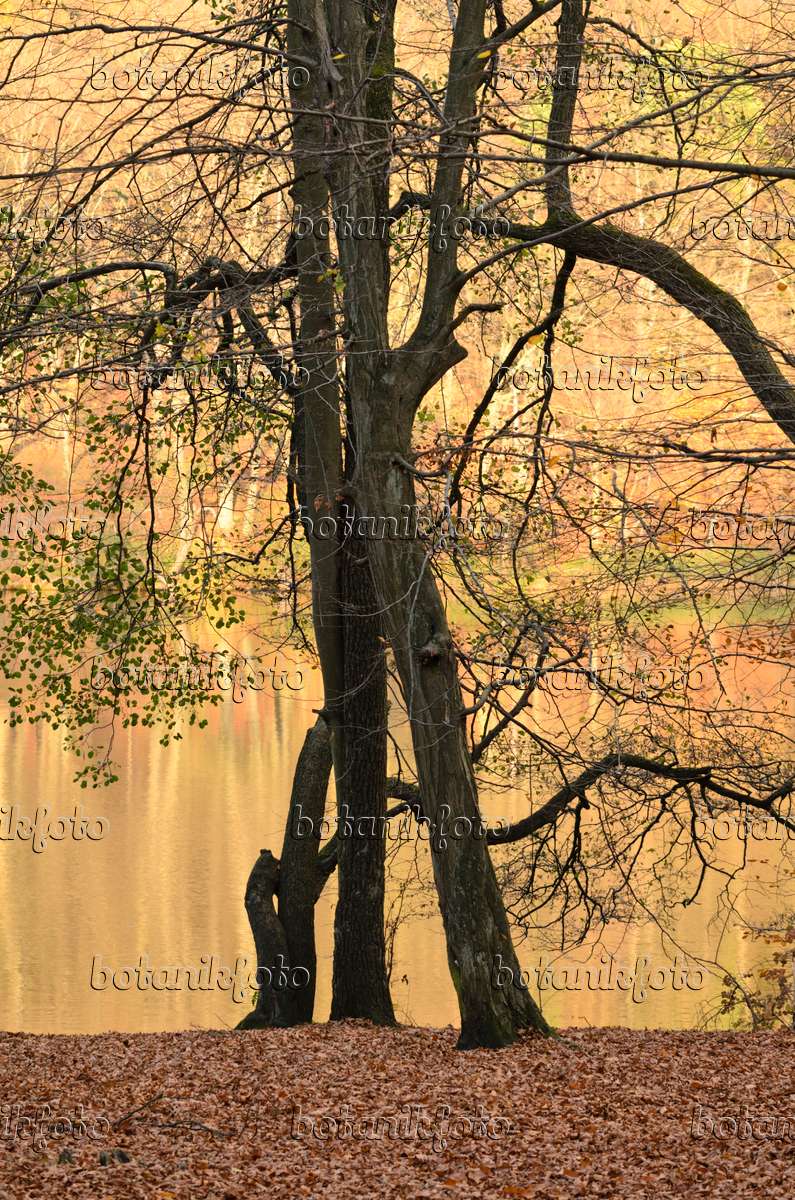This color photograph captures a serene, wooded scene in late autumn, marked by the warm, yellow glow of daylight. Central to the image are three large tree trunks that appear to intertwine, their branches sprawling in all directions, interspersed with a few remaining leaves. The foreground is a dense carpet of fallen leaves, reinforcing the fall setting. The primary tree stands in shadow, while a sunlit lake and distant white-barked trees, likely aspens, form a reflective, golden background. Multiple watermark overlays stating "Botanik Foto" are present across the image, marking it clearly as their proprietary work.